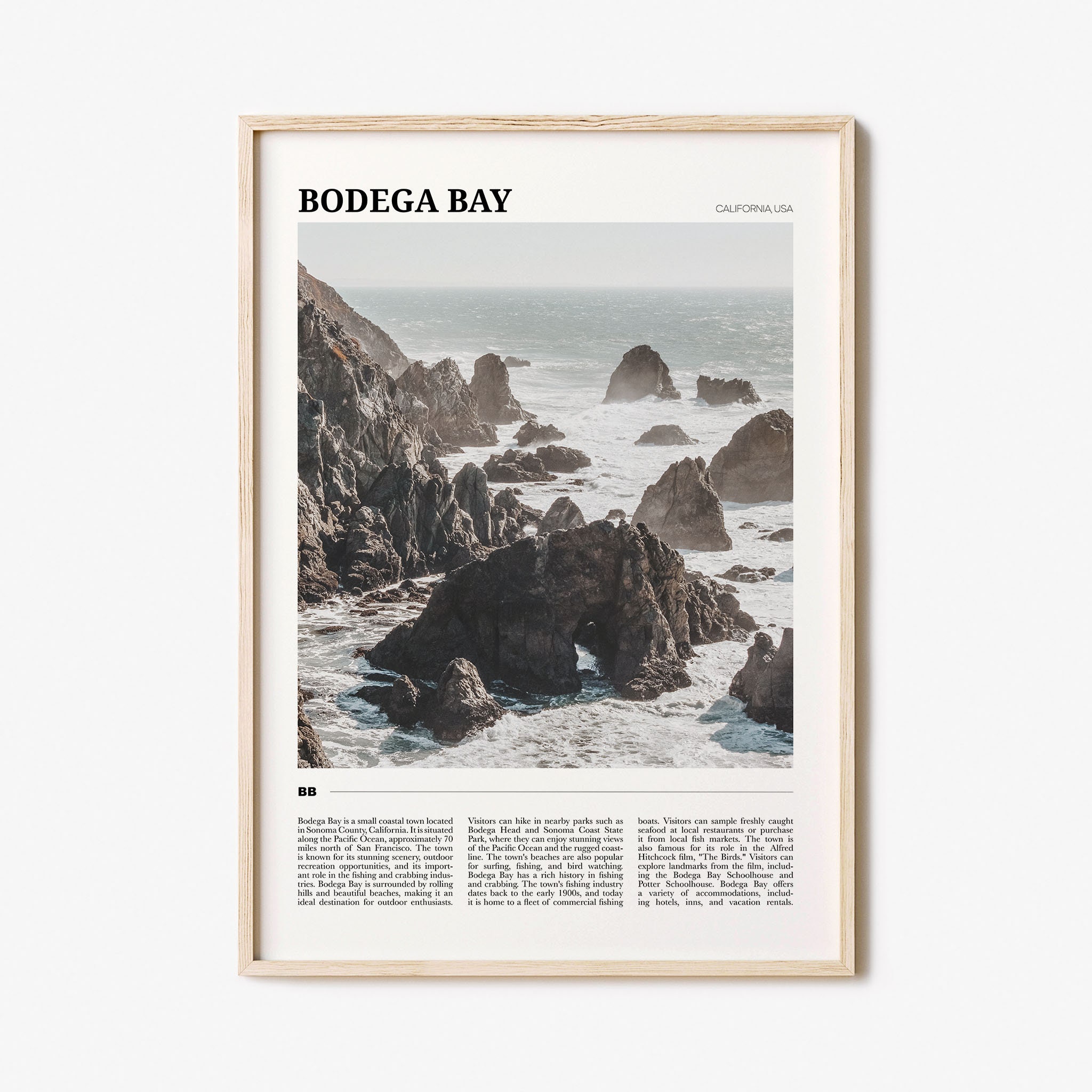This detailed caption for the image consolidates information from all three descriptions:

"The image is a framed photograph resembling a magazine page, depicting the scenic shoreline of Bodega Bay, California, USA. The page is bordered in brown and set against a light blue wall, and features 'Bodega Bay' in prominent black letters in the top left corner, with 'California, USA' to the right. The scene captures a misty, somewhat sunny day with a light gray sky dotted by sparse, gloomy clouds. A calm yet foamy ocean meets a rugged shoreline with numerous rocky outcroppings. On the left side of the image, a cliff descends into the water, and along the shore, waves crash against the rocks. Though there is additional text beneath the photograph, it is too small to read."